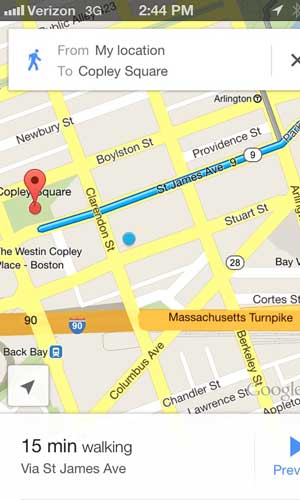The image showcases a navigation screen on a mobile phone. At the very top, a black bar displays essential information in white, including the signal strength with Verizon 3G, the time "2:44 p.m.," and a back icon. Below this, a white box contains navigation details with a blue icon of a walking person. It outlines a route from "My location" to "Copley Square," featuring an 'X' button on the far right to cancel the navigation.

The main section of the screen presents a map highlighting various streets in yellow against a gray background, indicating buildings. Key streets such as Newbury Street, Boylston Street, Clarendon Street, and Stewart Street are labeled. St. James Avenue is marked in blue, while the Massachusetts Turnpike (I-90) appears in orange at the bottom of the map.

Towards the bottom left of the screen, another white box shows a walking route, stating it will take "15 minutes via St. James Avenue." On the far right, a blue button labeled "Preview" with a right-pointing arrow allows for further route details. The overall layout provides a clear and detailed navigation guide.